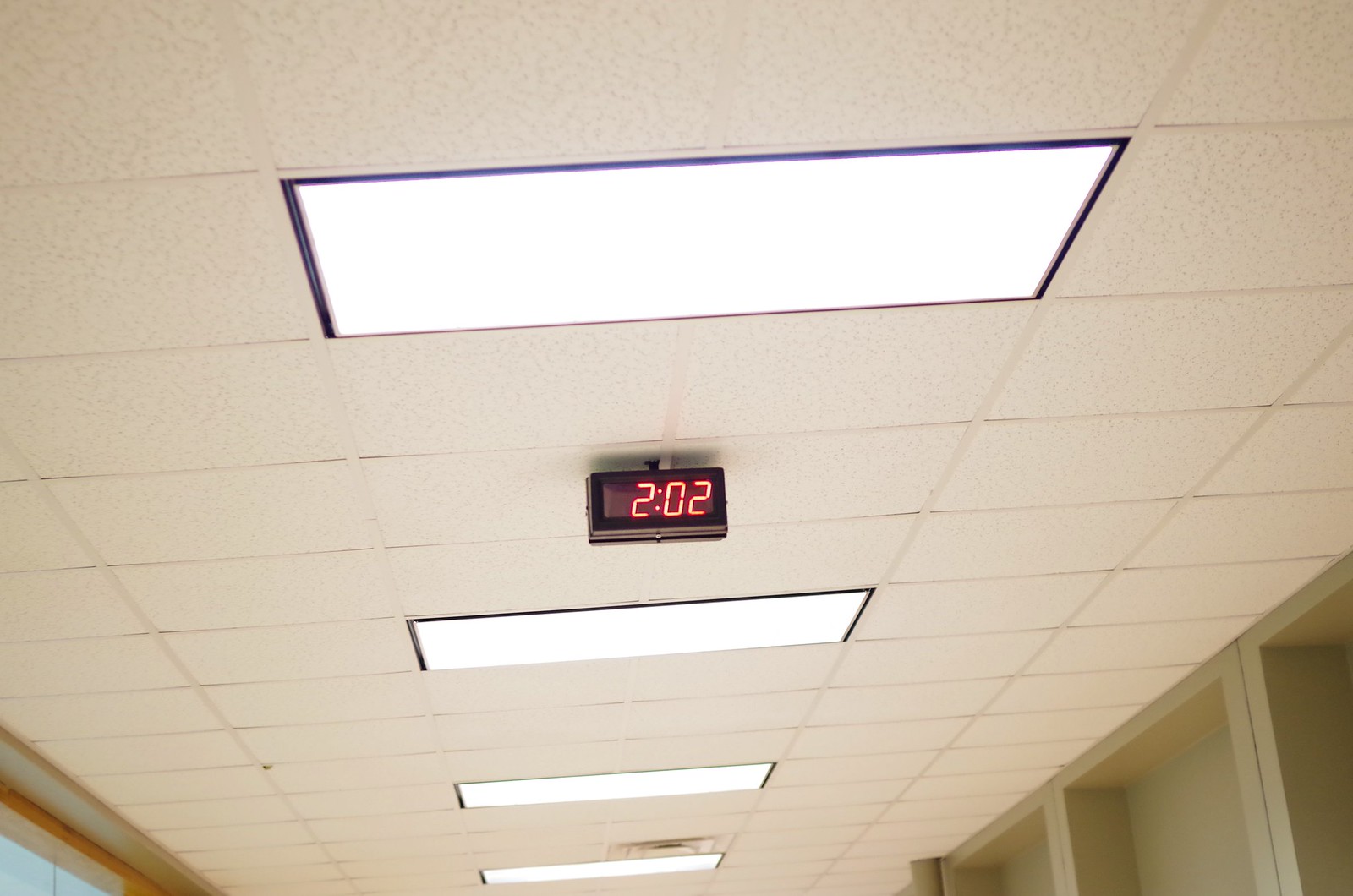This photograph showcases an expanse of a drop tile ceiling with a distinct sponge-like texture. There are six tiles aligned across the center of the image, while only three tiles are visible at the top foreground. The ceiling features four white fluorescent lights with metal trims around the edges, providing ample illumination. Positioned between the first and second light is a digital clock with black casing and brown trim, displaying the time 2:02 in bright red digits. Adding depth to the scene, a sliver of a tan wall is visible along both the right and left edges of the frame.